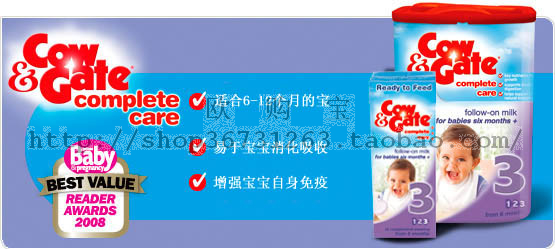This advertisement, set against a light purplish-blue background, features prominently the Cow and Gate Complete Care baby formula. In the top left corner, "Cow and Gate Complete Care" is written in red, accompanied by the "Baby and Pregnancy Best Value Reader Awards 2008" banner. Central to the ad are three check marks next to white text in Chinese characters, enclosed in red circles. To the right, the ad displays two packages of the Cow and Gate Follow On Milk for babies aged 6 months and older, showcasing a smiling baby and a large purple number 3. This ready-to-feed product aims to provide essential nutrition for growing infants.